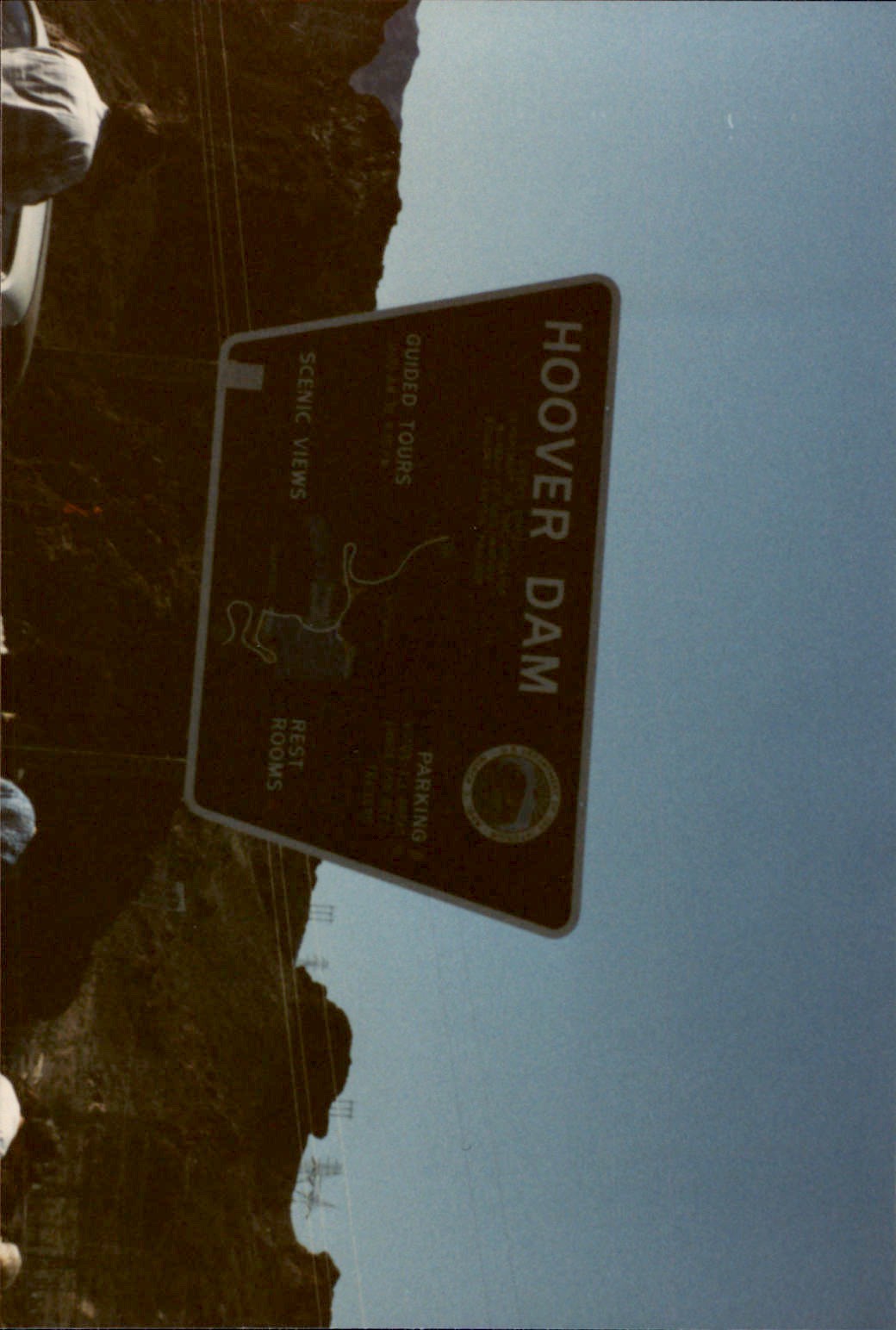The image depicts an old, slightly yellowed photograph taken at the Hoover Dam, with the picture oriented 90 degrees to the side. At the center of the image is a brown, white-trimmed sign with text that reads "Hoover Dam" and below it, "guided tours, scenic views, parking, and restrooms." The top-right corner of the sign features what appears to be a National Parks-like logo. In the foreground, there is a person visible from the waist up, wearing a white shirt. This individual seems to be near their parked car, located in the bottom left corner when viewing the image correctly. The backdrop includes greenish-brown rocky mountains, some with power lines spanning across them, suggesting proximity to the dam itself. Above, a clear, cloudless blue sky completes the scene, emphasizing the natural beauty of the setting. The overall ambiance suggests a roadside attraction captured in an era reminiscent of the 1970s or 1980s.